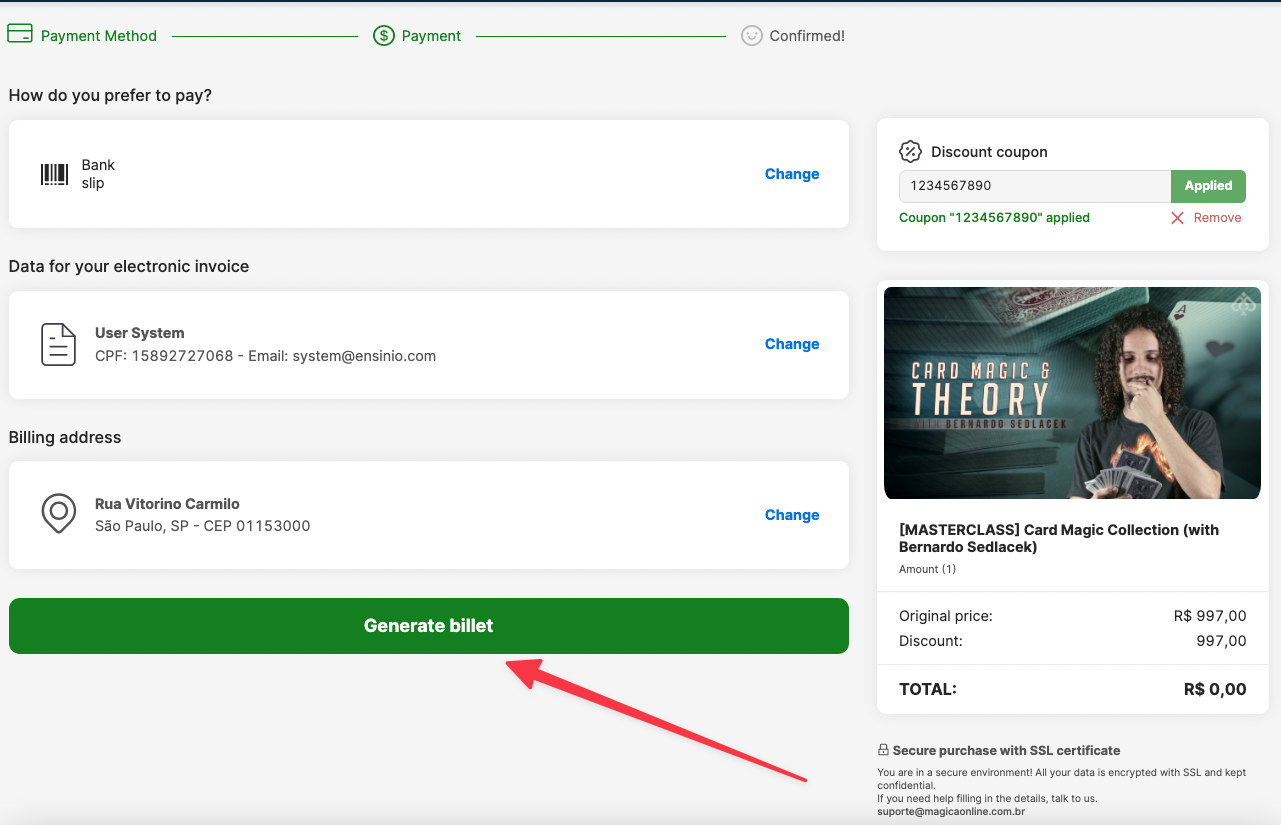Screenshot of a billing page for a card magic class featuring an image of Barnardo C. Dalek. In the bottom right corner, Dalek is depicted with a mustache, curly black hair, and wearing a black t-shirt, holding a deck of cards up to his face, next to the text "Card Magic in Theory with Barnardo C. Dalek."

At the top of the page, it shows the payment process with steps: "Payment Method," "Payment," and "Confirmed." Below this, it asks "How do you prefer to pay?" with an option to change the payment method, currently set to "Bank Slip."

Following that, there's a section titled "Data for your Electronic Invoice" and "Billing Address," both of which can be modified by the user. Below these sections, there's a prominent green rectangular button labeled "Generate Bill," indicating the next step.

At the top right of the image of Barnardo, there’s a section for a discount coupon. The coupon code "1234567890" is shown in the input bar with a green button labeled "Apply." The coupon application status is confirmed below with an option to remove the coupon if desired.

At the very bottom of the page, there's a note stating "Secure Purchase with SSL Certificate," indicating a secure transaction process.